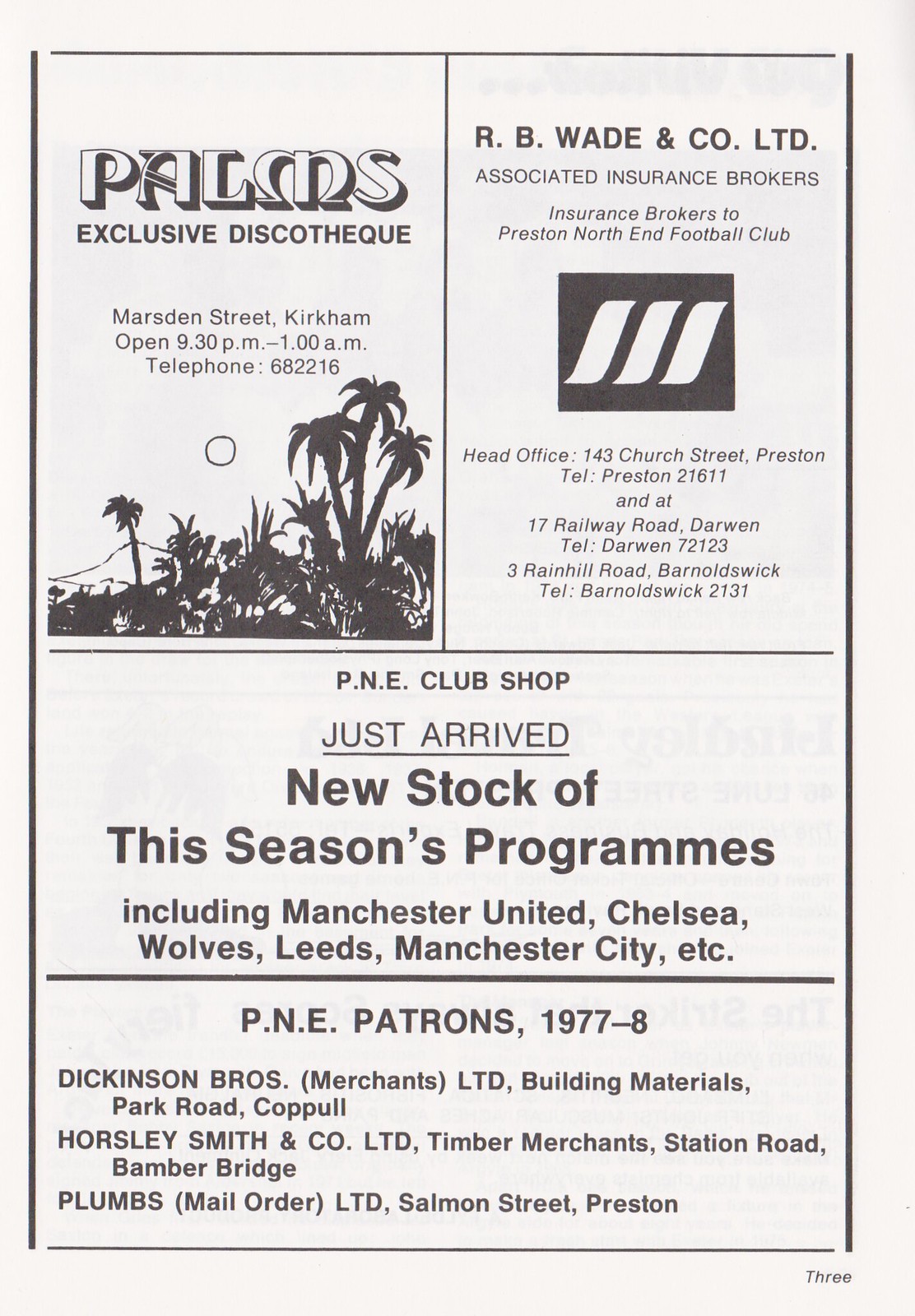The image is a detailed black and white flyer, structured like a page from a sports program, featuring four separate advertisements within distinct boxes framed by a solid black rectangle on a white background. 

The top left box advertises the Palms Exclusive Discotheque located on Marston Street, Kirkham, detailing its operating hours from 7:30 p.m. to 1:00 a.m. and providing a contact number, 682216. Adjacent to it, the top right box highlights RB Wade and Co. Ltd., insurance brokers associated with Preston North End Football Club, with offices at 143 Church Street, Preston (telephone: Preston 21611), and another at 17 Railway Road, Darwin. 

Other boxes include information about the P&E Club Shop's new stock of this season's programs featuring teams like Manchester United, Chelsea, Wolves, Leeds, and Manchester City, as well as other ads for Dickinson Bros, Limited (building materials), Horsley, Smith & Co. Ltd (timber merchants), and Plums Mail Order Ltd located on Salmon Street, Preston. The flyer appears to be from a local magazine or a sponsor-filled sports program, judging by its content and layout.